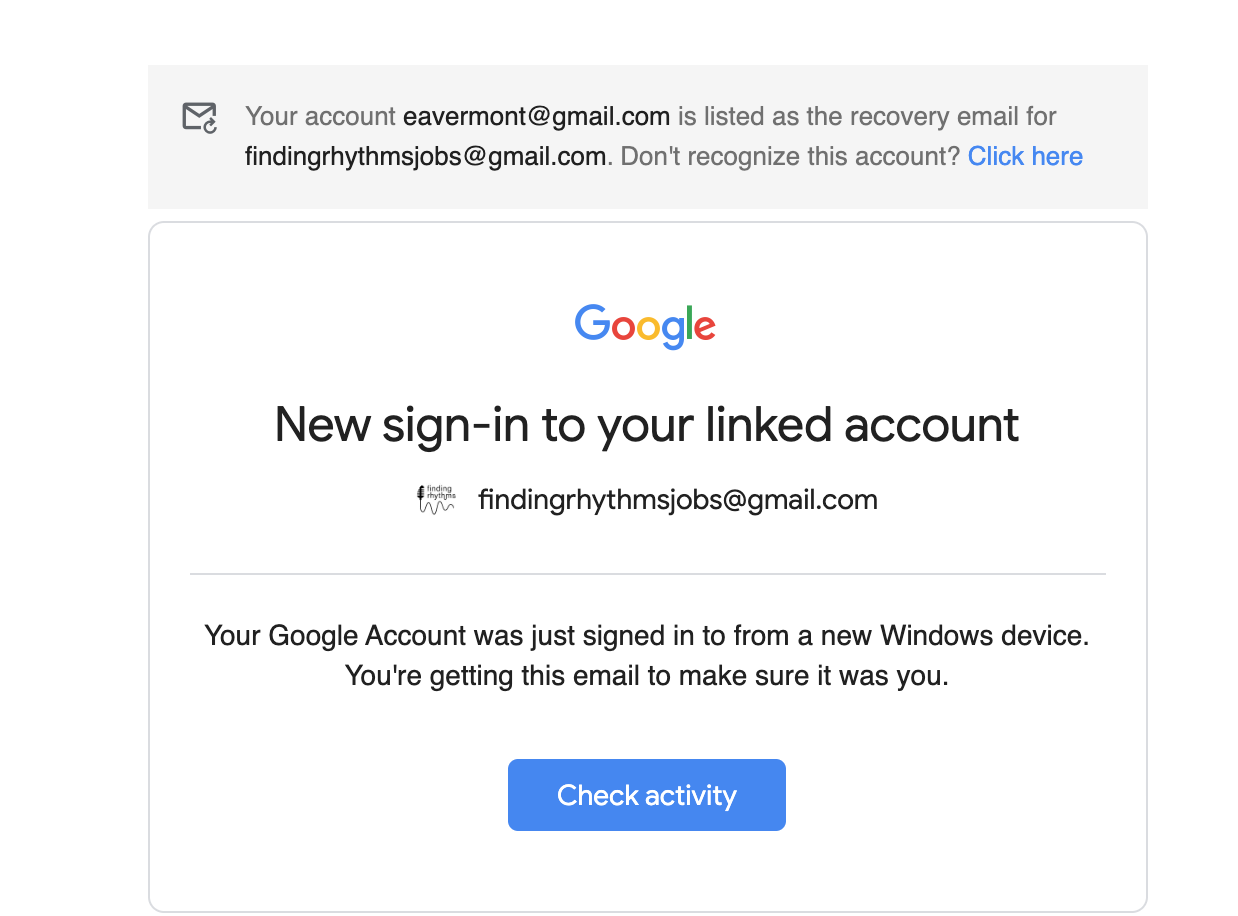The image features an email layout themed in various shades of gray and white. At the top of the email, a message indicates that the email address vermont@gmail.com is listed as a recovery email for the account findingrhythmsjobs@gmail.com. The message provides a prompt for the recipient to click a "Reminder" link if they do not recognize the account.

Below this message, there is a prominent, colorful Google logo consisting of a large blue "G," followed by red, yellow, and blue letters spelling out "oogle."

Midway through the email, there is a notification about a recent sign-in to a LinkedIn account associated with the email address findingrhythmsjobs@gmail.com.

At the bottom of the email, another message indicates that the Google account associated with findingrhythmsjobs@gmail.com was recently accessed from a new Windows device. This message is accompanied by a blue rectangle button labeled "Check Activity."

The email features subtle gray edges and a white background, with some additional text identifying this as part of Google's account recovery procedure.